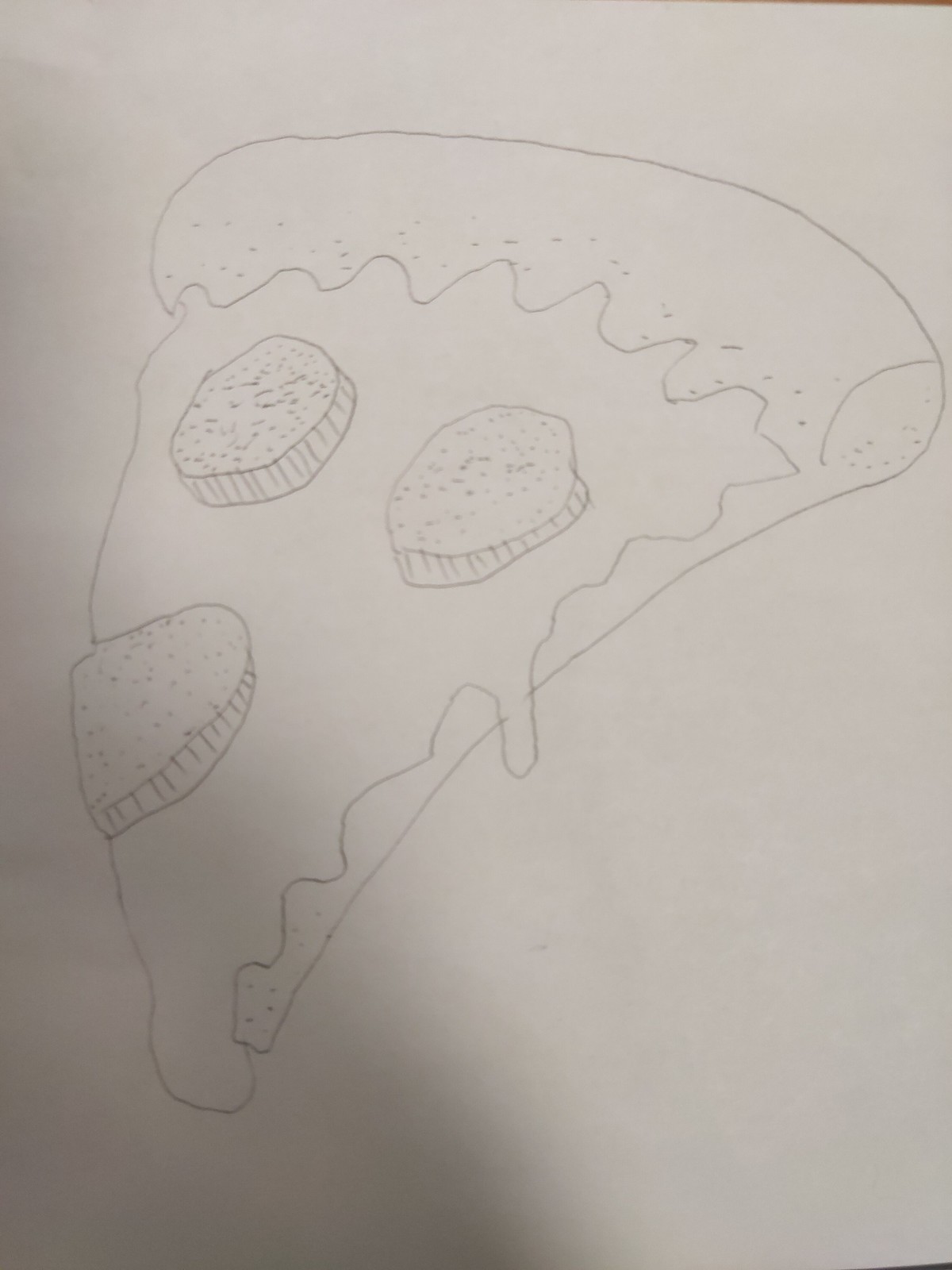The image displays a detailed pencil sketch on a square sheet of white paper. The paper is positioned on a surface that reveals a brown sliver, possibly a table or some other flat surface at both the top right and bottom right corners. The focal point of the drawing is a slice of pizza viewed from the side, capturing both the top and the profile. The crust is prominently visible at the top, rounded and textured, leading to the typical triangular shape extending downwards. The pizza is adorned with three pepperonis; two are fully visible as round discs while the third appears partially cut, suggesting it was sliced along with the pizza. The sketch meticulously depicts melted cheese that lavishly covers the pizza, with strands of cheese artistically portrayed as dripping over the sides and edges, enhancing the mouthwatering appeal of the slice.